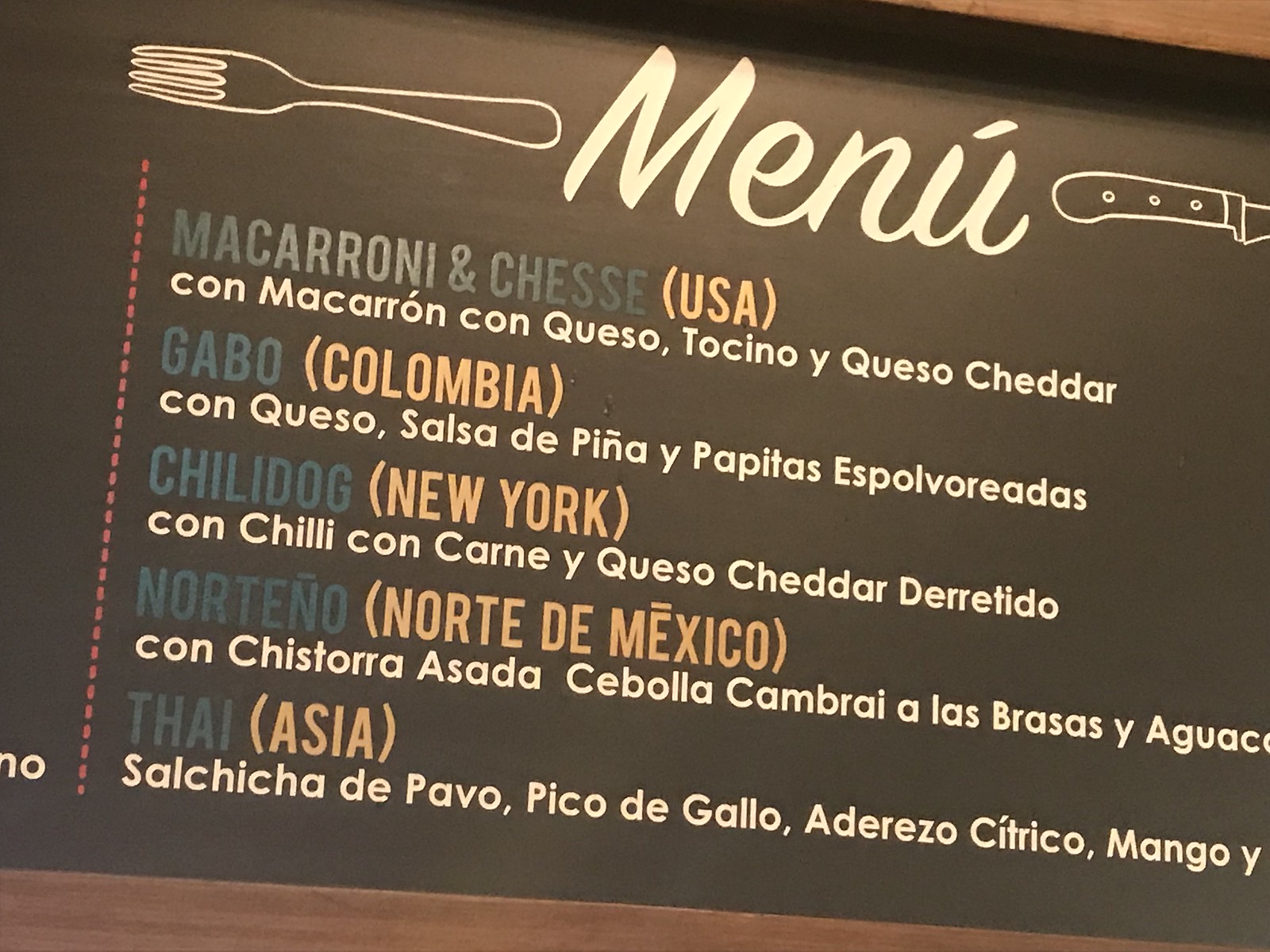The image captures a detailed view of a restaurant menu board mounted on a dark wooden frame. The board itself is a deep, rich brown, almost black, providing a striking contrast with the text and icons. At the very top, the word "Menu" is prominently displayed in bold white letters. Flanking the title, a white silhouette of a knife is depicted on the right side, and a fork on the left, giving a touch of culinary elegance.

Below the title, the menu lists several international dishes, with their names suggesting their regional origins. The first item is "Macaroni and Cheese, USA," followed by what appears to be the same dish name written in an unidentifiable language. Next is "Gabo, Colombia," then "Chili Dog, New York," moving on to "Nortino, Norte de Mexico," and concluding with "Thai, Asia."

A thin, dotted red line runs vertically down the left side of the board, hinting at a possible division of different menu sections, though this segment is not visible in the image. The color scheme consists of various shades of gray, dark browns, white, and a muted peach hue, lending the menu a sophisticated yet warm aesthetic. The photo is a close-up, focusing exclusively on this particular section of the menu, capturing the details and textures clearly.